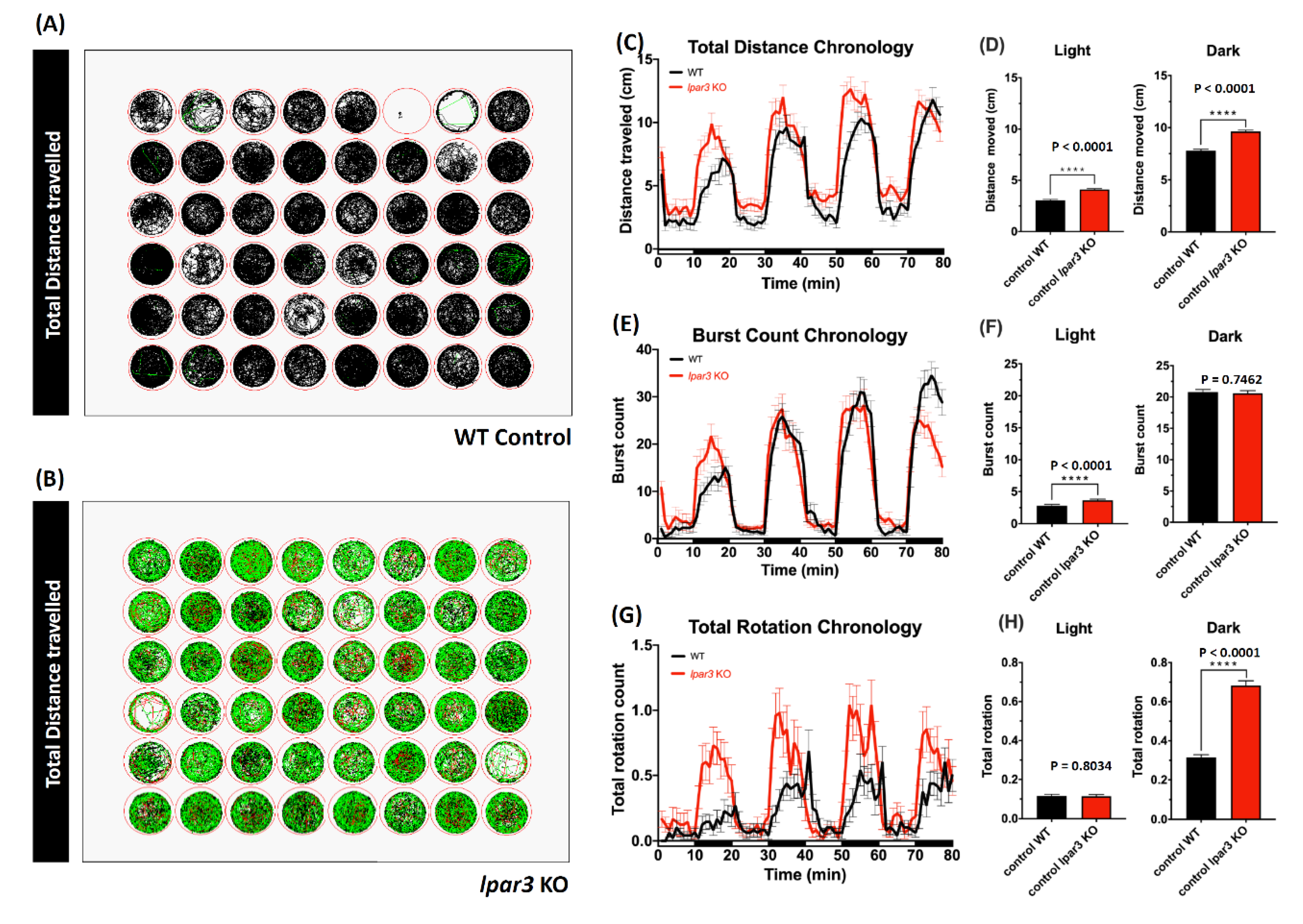The image displays a variety of infographics and diagrams organized into three main sections. On the far left, there are two grids labeled WT Control (top) and IP3K/IPAR 3KO (bottom), both titled "Total Distance Traveled." Each grid consists of 36 circles randomly filled in, with the top grid featuring predominantly black circles and the bottom one predominantly green. Both grids have red lines around certain circles.

In the central section of the image, there are three line graphs representing different types of chronologies: "Total Distance Chronology" (top), "Burst Count Chronology" (middle), and "Total Rotation Chronology" (bottom). These graphs feature black and red lines that fluctuate significantly, indicating variations over time.

On the far right, the image includes six bar graphs grouped in pairs. These bar graphs display data for light and dark conditions and feature black and red bars.

The overall image appears to visualize complex data related to travel distances, various chronologies, and environmental conditions, although the exact context remains unclear.